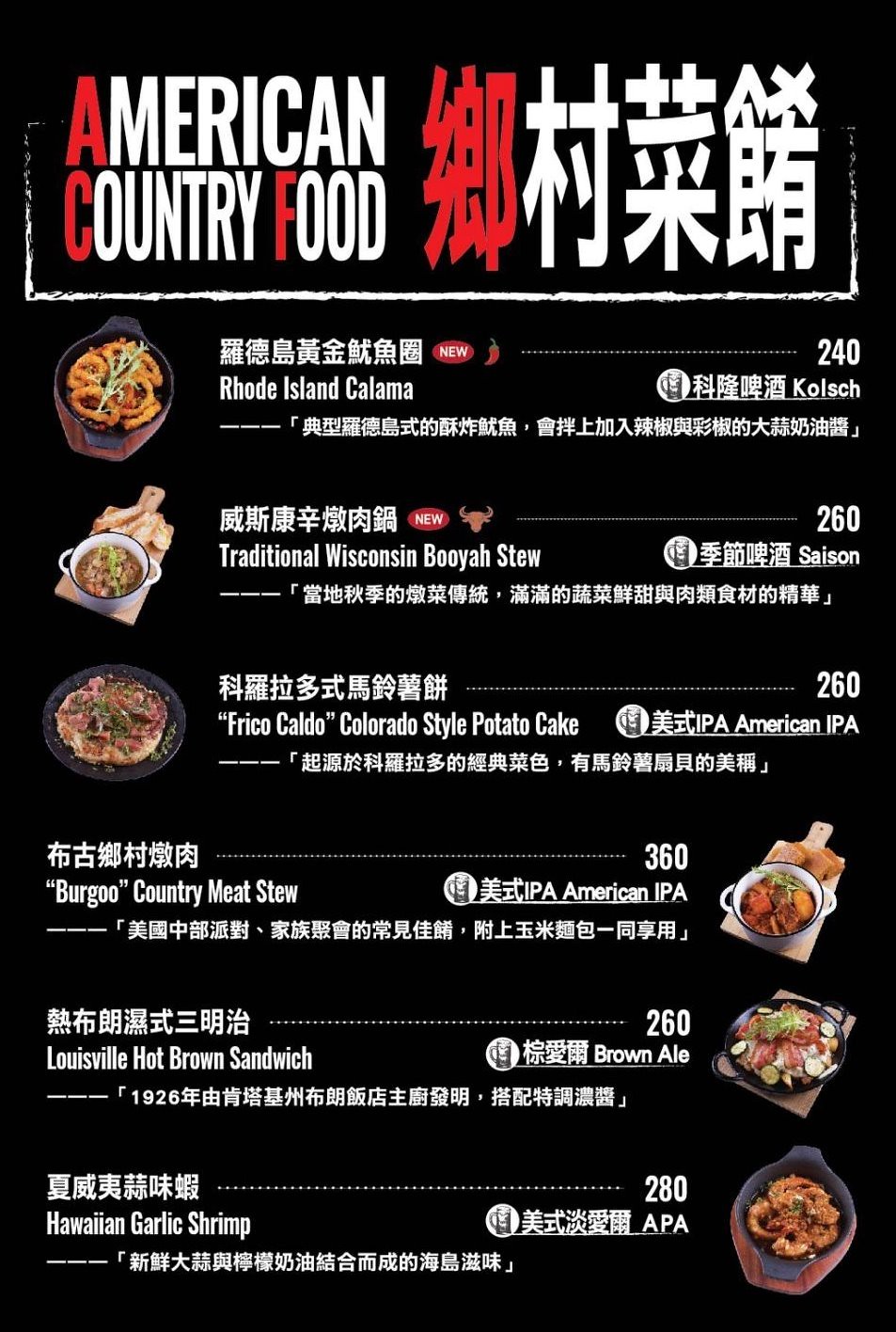This poster, presumably promoting Chinese cuisine, features a visually striking design dominated by a black background with red and white accents. The only English text prominently displayed reads "American Country Food," with the initials "A," "C," and "F" in bold red, contrasting with the rest of the white text. Surrounding the English phrase are red and white Chinese characters, adding to the cultural fusion theme of the poster.

The poster features an array of food photographs, each distinctively presented. The first image showcases a hot plate filled with what appears to be onion rings, accompanied by the phrase "Rhode Island Calamari." Next, an image of a cutting board with pieces of bread and a mug of soup is labeled "Traditional Wisconsin Booyah Stew."

Another dish, possibly a pizza with sushi elements, is displayed on a black plate and identified as "Frico Caldo Colorado Style Potato Cake." The layout then shifts, with photographs now positioned on the right side. One such image depicts a cutting board with bread and stew, titled "Burgoo Country Meat Stew."

Additional dishes include a "Louisville Hot Brown Sandwich" shown on a black plate, and "Hawaiian Garlic Shrimp" presented in a black dish. The overall color scheme of black, red, and white, combined with the blend of photographed dishes and their culturally rich names, create an intriguing and detailed visual narrative that bridges American country food with Chinese influences.